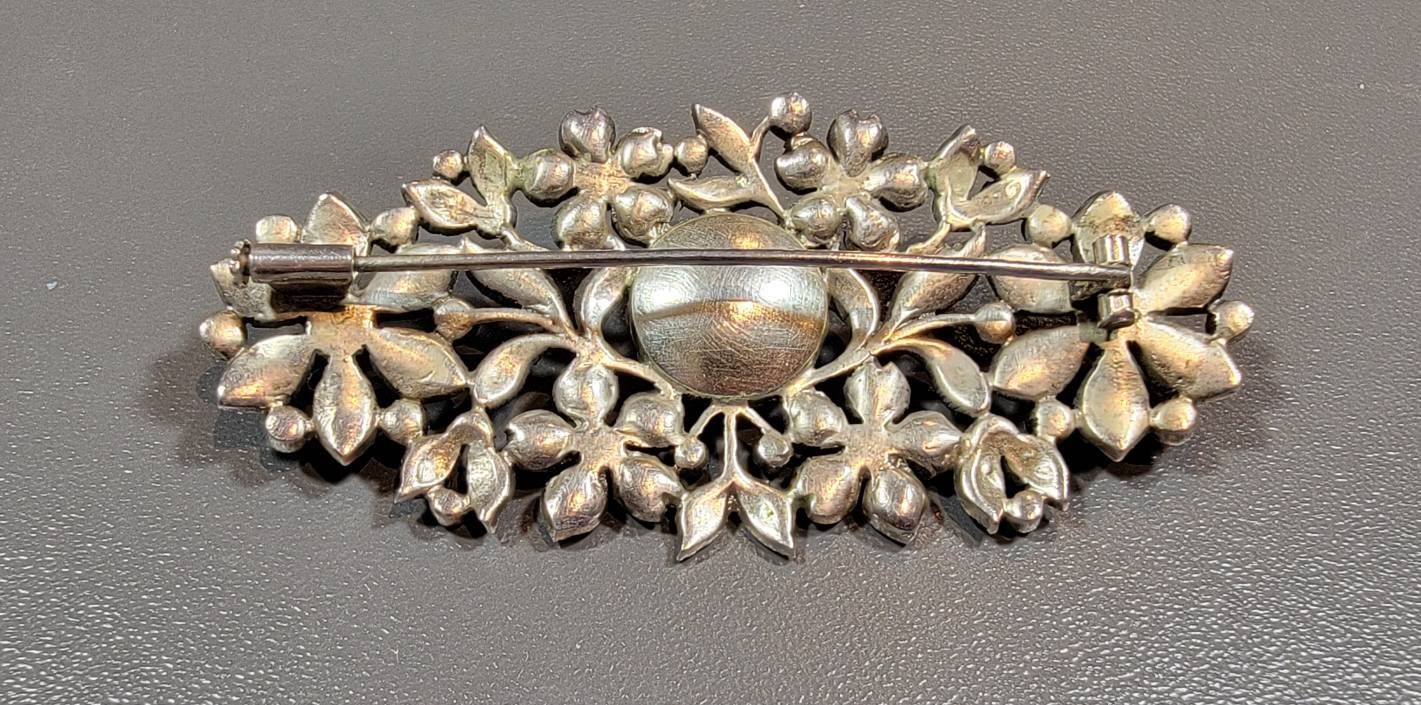The photograph captures the reverse side of a vintage brooch, prominently displaying its pin and locking mechanism, designed to secure it to clothing. The brooch is made of aged silver metal with a hint of yellowing, enhancing its vintage appeal. The intricate design reveals an oval shape adorned with delicate metallic flowers, leaves, and vine-like engravings, evoking a botanical motif reminiscent of classic Hawaiian jewelry. At the center, there appears to be a smooth jewel or sphere, adding a focal point to the floral arrangement. The entire piece rests on a textured gray surface, perhaps leather or vinyl, which complements the brooch’s detailed craftsmanship and adds a subtle contrast to the metallic sheen and grainy texture.